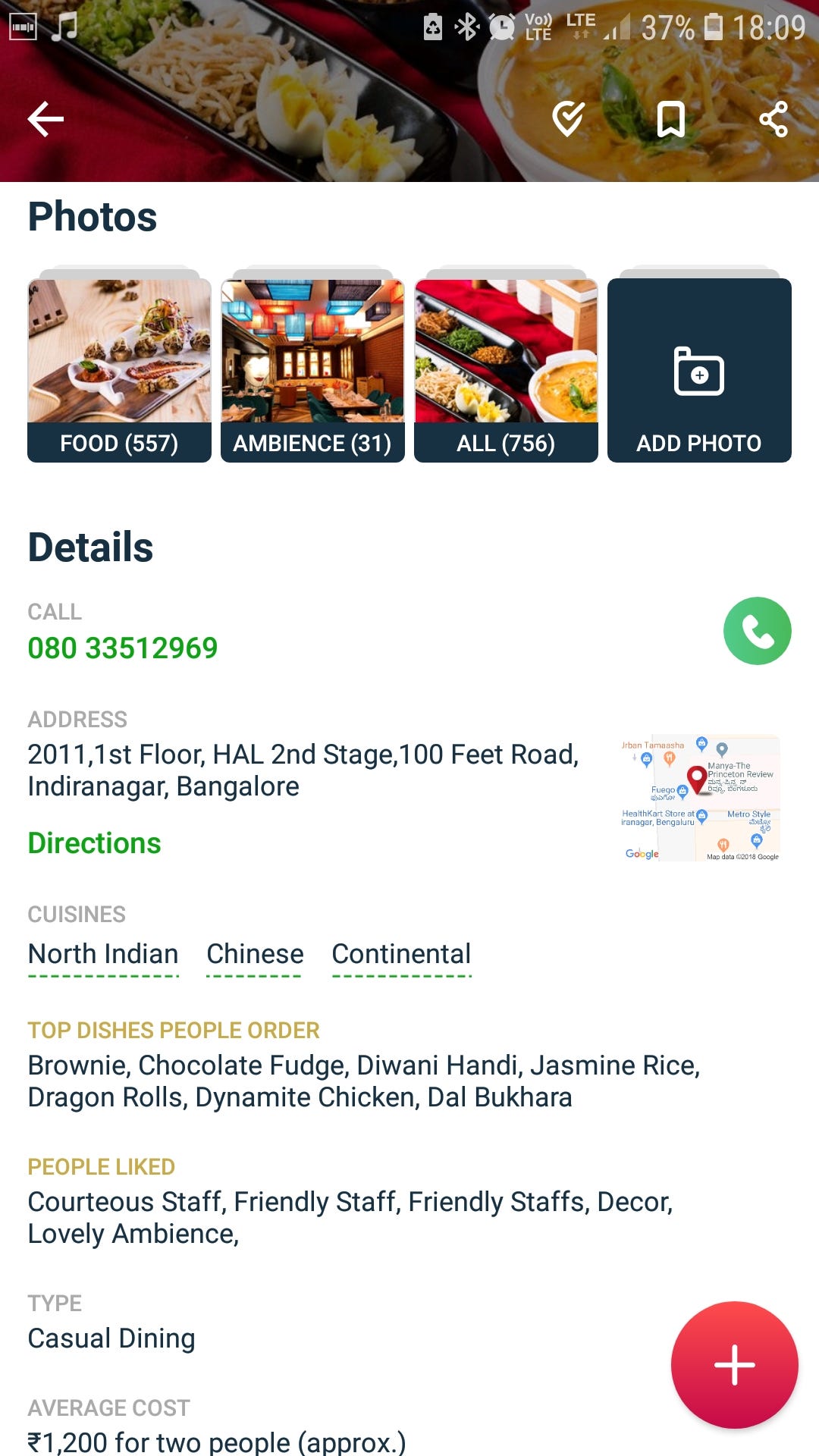A detailed phone screenshot showing a plate of Chinese food, featuring rice and dumplings. The app interface displays a 'Photos' section with four categories: 'Food' (557 photos), 'Ambience' (31 photos), 'All' (756 photos), and 'Add Photo'. Below this, the interface offers options like 'Details', 'Call' with a green phone icon and the number 080-3351-2969, and 'Address' listed as 2011, First Floor, HAL Second Stage, 100 Feet Road, Doddanekkundi, Bangalore. The address section includes a 'Directions' hyperlink. The 'Cuisine' section mentions North Indian, Chinese, and Continental dishes, while 'Top Dishes People Order' include brownie, chocolate fudge, diwani handi, jasmine rice, dragon roll, dynamite chicken, and dal bukhara. A red circle with a plus mark is also visible on the interface.